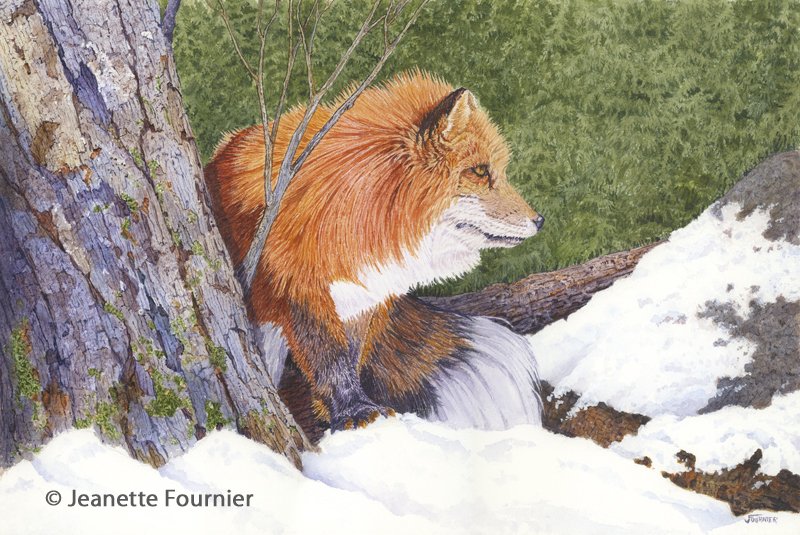The image depicts a very lifelike painting of an adult red fox set in a snowy forest landscape. The fox is positioned almost leaning against a moss-covered brown tree trunk located on the far left of the image, with several twigs and branches extending around it. The fox’s red fur contrasts with its distinctive black-rimmed brown eyes, black ears, black-tipped nose, and partially white muzzle and chest. One of its front paws, which is black and brown, is visible resting in the snow. Its tail is a mix of brown and black with a long white tip, curling gracefully behind.

The background comprises lush green foliage, giving a sense of a dense forest, with scattered branches, some of which appear to be fallen. The forest floor in the foreground is thickly blanketed with snow, and directly to the fox's right, there is a gray and brown rock partially covered with melting snow.

In the bottom left corner of the image, the name “Jeannette Fournier” is inscribed in gray font accompanied by a copyright symbol (©). There is also what appears to be an autograph signature “Jay Forner” on the bottom right corner, implying the artist's name. This careful attention to detail in both the fox and its natural surroundings creates an immersive, serene atmosphere, characteristic of a meticulously detailed painting.